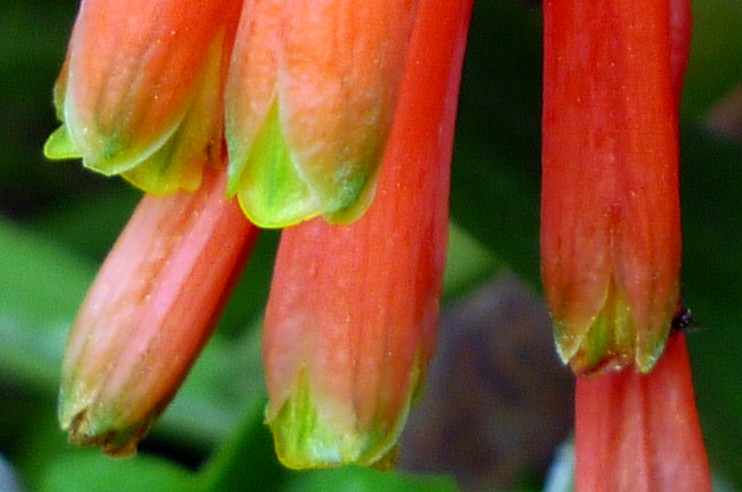In this close-up photograph, you see six long, tubular flower buds hanging upside down. These buds are primarily light reddish in color, with their tips tinged in green. The shot is extremely detailed, focusing on the vibrant, unopened flowers while the background remains artfully blurred. Notably, the flowers show various stages of blooming; some are slightly opened, revealing where the petals would separate, while others remain tightly closed. An intriguing detail is the presence of a fly trapped within one of the buds, partially visible. The overall effect of the image is striking, drawing attention to the intricate details and vivid colors of the buds against the soft, out-of-focus green background.